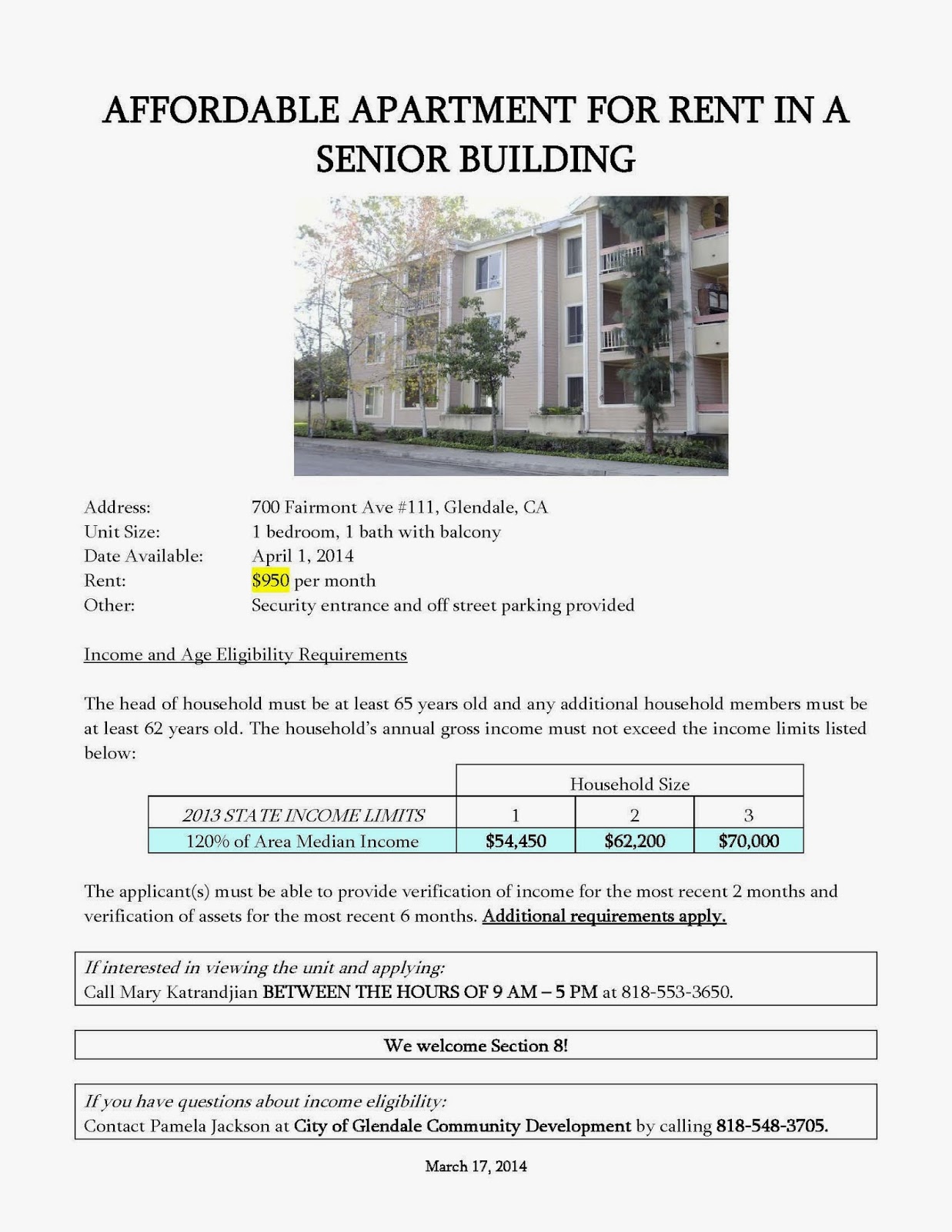**Affordable Apartment for Rent in Senior Building**

**Description:**

A well-maintained senior apartment at 700 Fairmont Avenue, No. 111, Glendale, California is now available for rent. The listing is presented on a gray background with predominantly black text interspersed with bold and highlighted sections for emphasis.

**Rental Details:**
- **Address:** 700 Fairmont Avenue, No. 111, Glendale, California
- **Unit Size:** One bedroom, one bath with a balcony
- **Available Date:** April 1, 2014
- **Rent:** $950 per month (highlighted in yellow)

**Features:**
- Security entrance
- Off-street parking provided

**Eligibility Requirements:**
- **Age:** The head of household must be at least 65 years old; all additional household members must be at least 62 years old.
- **Income:** The household’s annual gross income must not exceed the income limits listed below:
  - One person: $54,450 (120% of the 2013 state income limits)
  - Two people: $62,200
  - Three people: $70,000
   
   (Income figures highlighted in blue)

Applicants must provide:
- Verification of income for the most recent two months
- Verification of assets for the most recent six months
- Additional requirements may apply

**Contact Information:**
- **Interested applicants** should call Mary Kandandram between 9 a.m. and 5 p.m. at 818-553-3650.
- **For questions about income eligibility,** contact Pamela Jackson at City of Glendale Community Development at 818-548-3705.

**Additional Information:**
- Section 8 vouchers are welcome.
- Listing date: March 17, 2014

**Visual Description:**

The top section of the image emphasizes the availability of an "Affordable Apartment for Rent in a Senior Building" in bold black font. Below that, a photograph showcases a light tan apartment building with white windows and green shrubbery. The subsequent sections provide detailed rental and eligibility information in black text, accented with yellow and blue highlights for important details.